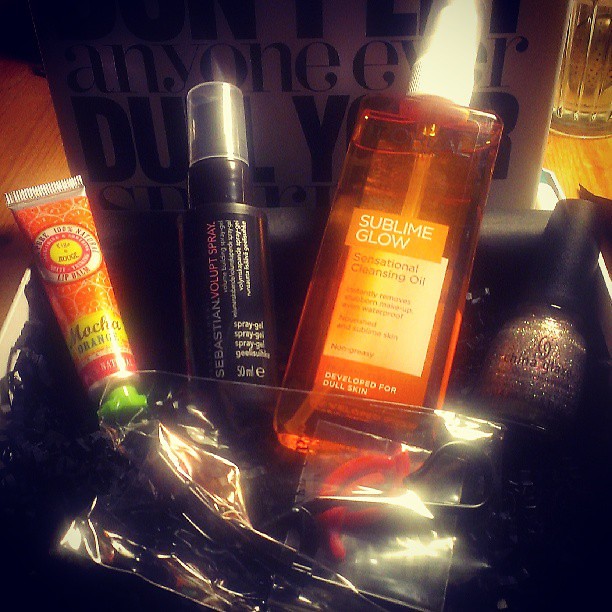In this photograph, a collection of various body care products is displayed in a white cardboard tray with a black paper lining. The items are neatly arranged from left to right, fanned out for visibility. The image has a hazy, blurry quality, as if viewed through a greasy lens, which lends a soft glow to the scene.

Starting from the left, there is an orange tube labeled "Mocha Orange", featuring a green screw cap. Next to it, slightly to the right, stands a black cylindrical spray bottle with a clear plastic cap, identified as "Sebastian Volupt Spray". To its right, there's an oval-shaped transparent bottle filled with orange liquid, labeled "Sublime Glow Sensational Cleansing Oil" and described as being developed for dull skin. Following this, there's a bottle of China Glaze nail polish with a sparkly, metallic silver content and a black screw cap.

In front of these items, a plastic, transparent packet can be seen, holding an unspecified product, possibly hair clips, partly obscured by a glare from the camera flash. The tray is set on a wooden table which is barely visible at the upper left and right edges of the image. In the background, a poster with partly obscured text hangs on the wall. The legible portion reads, "anyone ever du something ly," which might be part of the phrase "dull your style".

Additionally, in the upper right corner of the image, part of a drinking glass is visible, adding a subtle context to the setting.